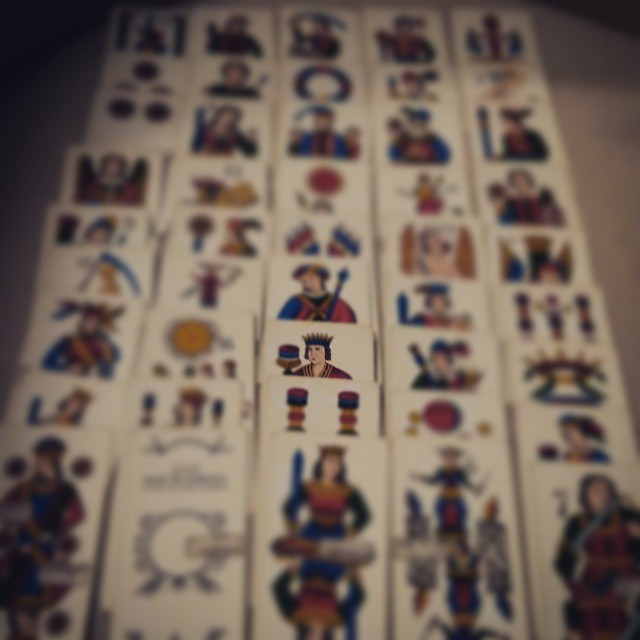The image showcases 40 cards arranged in a 5 by 8 grid on what appears to be a brown tabletop or carpet. These cards resemble playing cards in size, but they do not feature traditional suits like diamonds, clubs, hearts, or spades. Instead, they predominantly display various images and colored shapes.

The cards in the first and the last five rows are blurry, as are all the cards except for the middle card in the second row and the middle card in the third row. The middle card of the third row distinctly features an illustration of a king, while the card directly in front of it shows a collection of colored shapes. 

The overlapping arrangement limits the view of each card, with only the front row cards fully visible. Most of the cards exhibit pictorial representations rather than typical playing card symbols, adding to the uniqueness of the set.